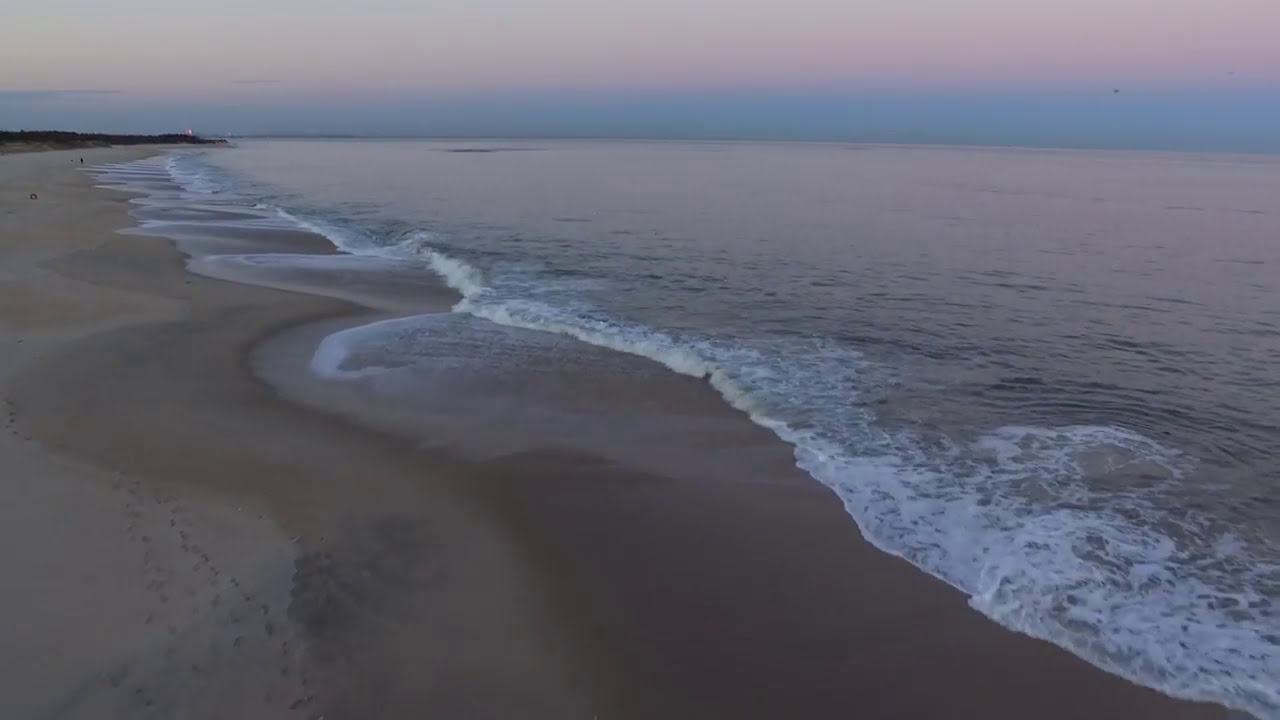This photograph, captured from a large aerial view, depicts a serene beach scene illuminated by low light, suggesting a sunset or overcast ambiance. The sky at the top of the image transitions from a light blue to a pastel reddish-orange before merging into a darker blue as it meets the horizon. The dark-colored ocean occupies the right side, with white waves rushing up to the shore. The sandy beach, varying from grayish-tan to darker wet areas, stretches across the left and bottom. Noticeable in the bottom left are footprints imprinted in the dry sand. In the distance, a patch of vegetation, possibly trees or grass, is visible on raised land that extends toward the sea as a small peninsula or island. Additional details include tiny silhouettes of people walking along the shore, and the overall scene appears misty, adding a moody, atmospheric touch to the photograph.